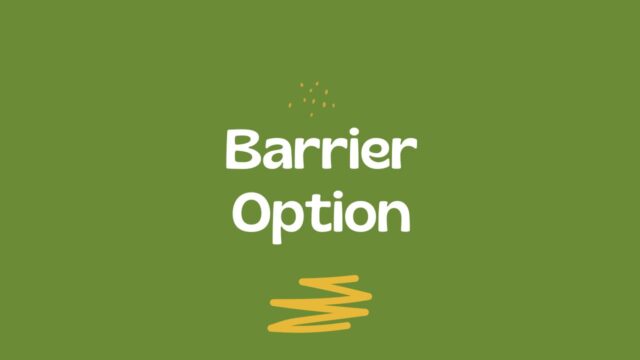The image is a rectangular green poster with a light olive green background. At the center, in bold white font, the word "Barrier" is prominently displayed, followed underneath by the word "Option." Beneath "Option" is a thick, zigzagging yellow line extending from top to bottom between the letters P and O. Above the word "Barrier," near the top of the image, is a series of small yellow dots arranged in a speckled, starburst pattern. The overall design features a simple color scheme of white for the text and yellow for the decorative elements against a pale green backdrop, possibly representing a logo or sign for the company named "Barrier Option."